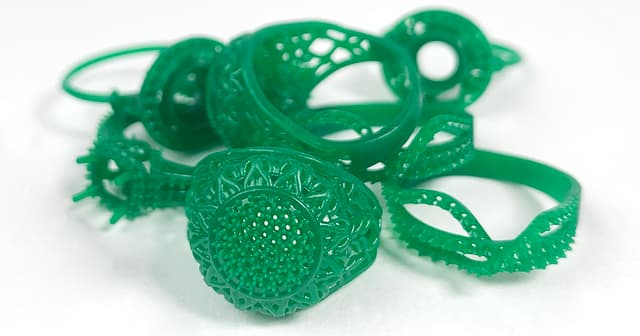The photograph showcases a close-up of several green rings, intricately arranged in a haphazard pile on a white surface with a white background. Each ring, exhibiting a glossy jade color, varies in size and style. The designs include one resembling a class ring adorned with the top of a sunflower, another composed of three rings that intertwine, and others with unique floral patterns. The material of the rings is ambiguous, appearing either as glossy jade stone or recycled plastic. These rings, free of any other metals, diamonds, or stones, cast faint shadows on the surface beneath them, adding depth and an element of mystery to the cluster. The overall arrangement presents a striking display of green, intertwined jewelry pieces.